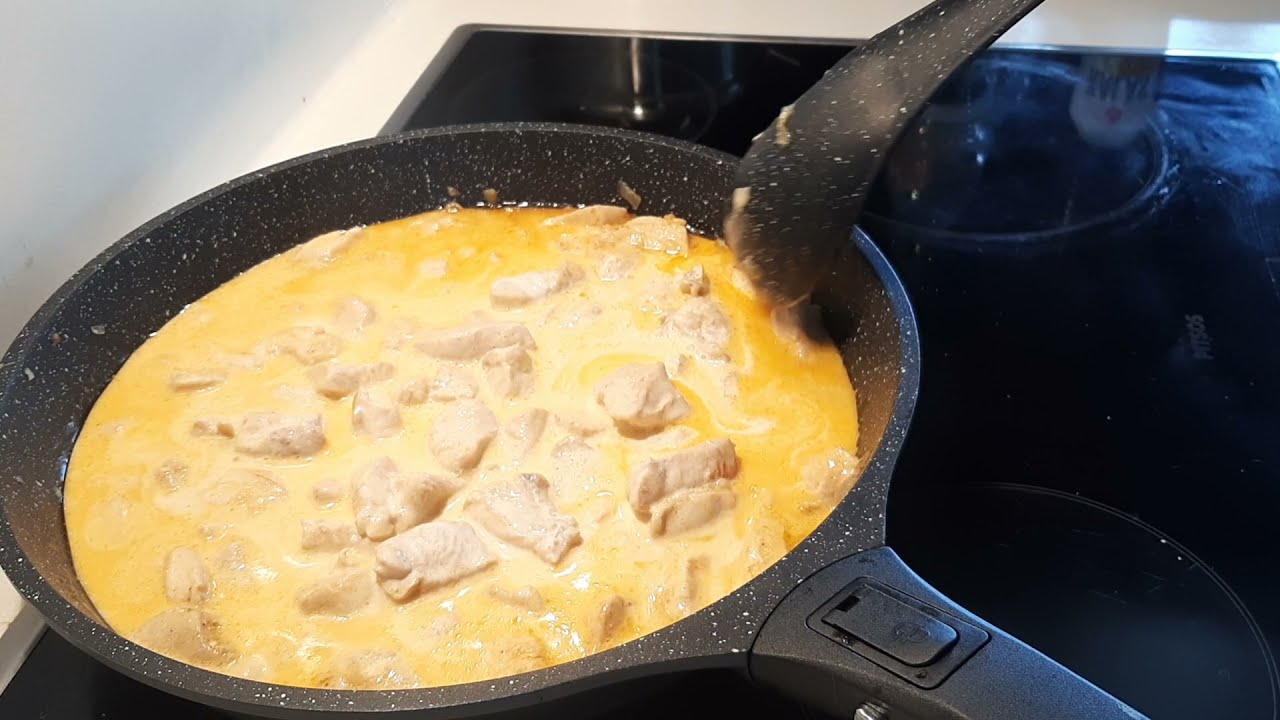In the image, we see a detailed scene of someone cooking in a kitchen. The focal point is a circular black pan with a plastic handle and a metallic rim, featuring white specks all over it. This pan is situated on a shiny, black, flat glass stove top. Inside the pan, pieces of chicken are being cooked in a vibrant yellow sauce, possibly a curry or egg-based mixture. The pan is positioned slightly towards the bottom left of the image's center. From the top right, a black spoon with matching white specks is actively stirring the contents of the pan. The setting appears to be an intimate kitchen environment, suggesting the preparation of a meal. The dominant colors in the scene are yellow, black, white, tan, gray, and silver, creating a visually engaging cooking moment.